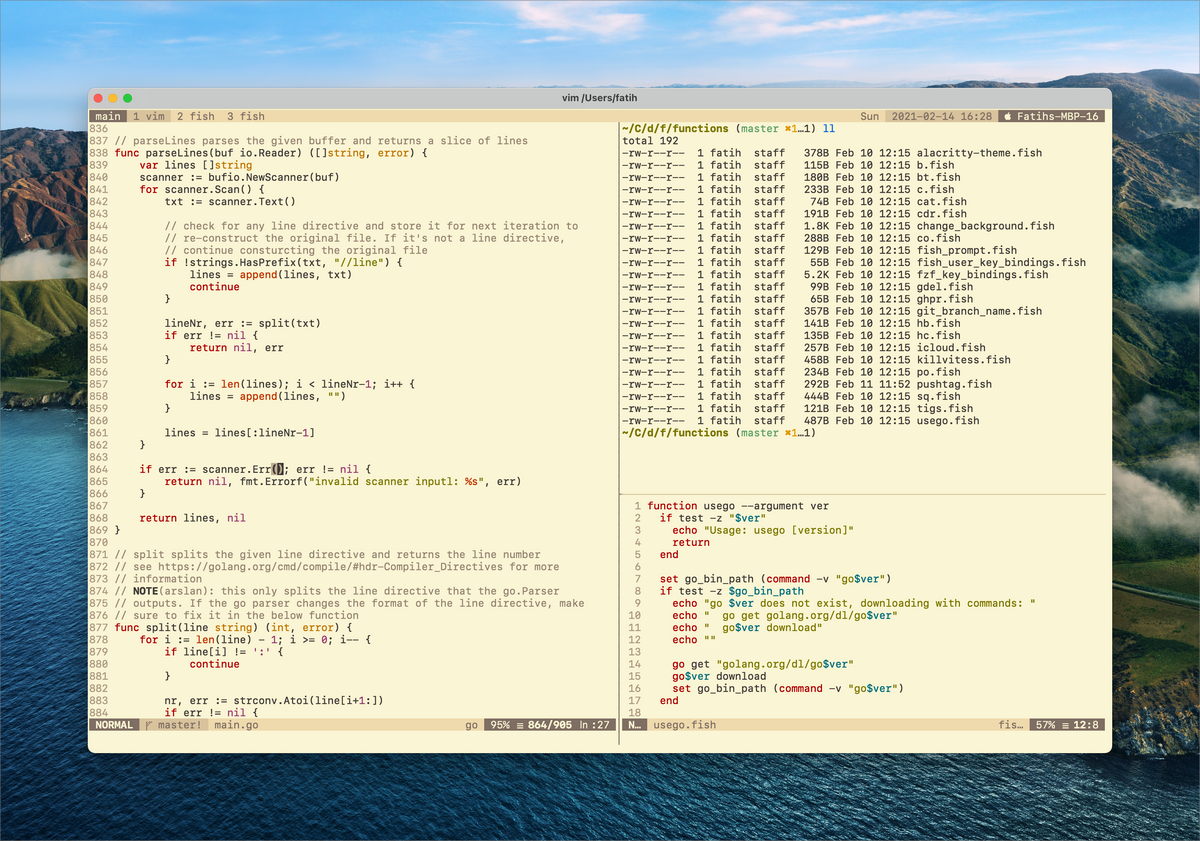The image is a detailed screenshot of a Mac computer screen, showcasing an open coding interface. The screen clearly belongs to a Mac operating system, identifiable by the characteristic three dots—red, yellow, and green—at the top left corner of the coding window. The coding interface itself is set against a scenic wallpaper of mountains and the ocean. The code, which appears in various colors—black, green, red, and blue—is displayed on a cream background with lines of text that include references to "vim/users/faith" and several mentions of "Faith Staff." The date on the screen shows Sunday, February 14, 2021, at 4:28 PM, and the battery icon indicates that the laptop is 67% charged.